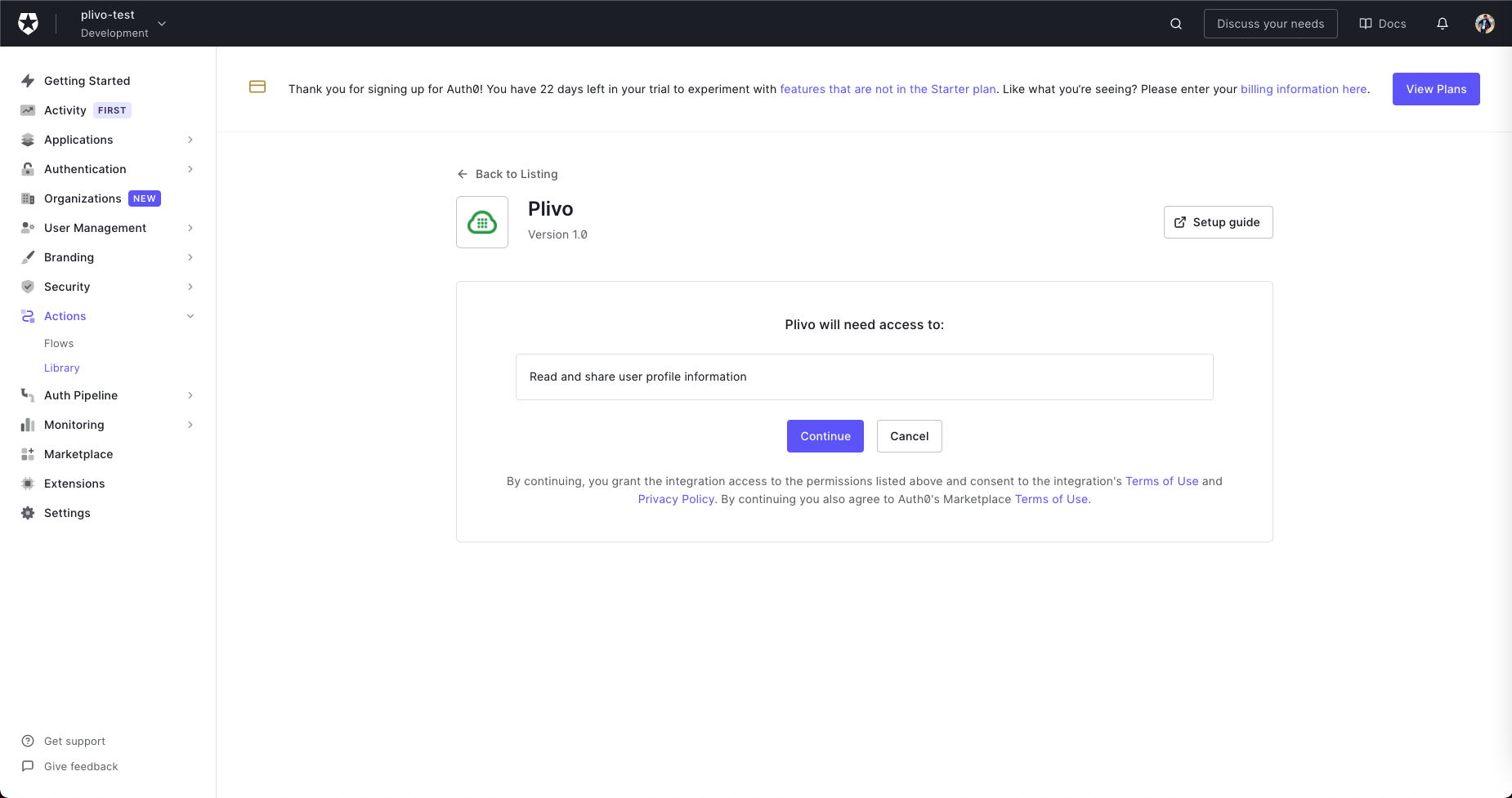The webpage interface prominently displays a black navigation bar at the top, branded with "PrevoTest." This bar includes a dropdown labeled "Development," a search bar with the prompt "Discuss Your Needs," a "Docs" section, a notification bell icon, and a user profile icon. Below this, a series of detailed tabs is available: Getting Started, Activity, Applications, Authentication, Organizations, User Management, Branding, Security, Actions, Auth Pipeline, Monitoring, Marketplace, Extensions, and Settings.

The main content of the page features a welcoming message: "Thank you for signing up for OTHO. You have 22 days left in your trial experiment with features that are not in the starter plan." Users are encouraged to provide their billing information via a purple "View Plans" button. 

A navigation cue is available with a "Back to Listing" link accompanied by a small gray backward arrow. An icon of a cloud with green dots indicates "Prevo version 1.0."

A "Setup Guide" section provides essential information, noting that "Prevo will need access to read and share user profile information." Users can proceed by clicking the purple "Continue" button or opt-out with the white "Cancel" button.

This detailed interface offers comprehensive navigation and prompts to guide users through managing and upgrading their PrevoTest experience.